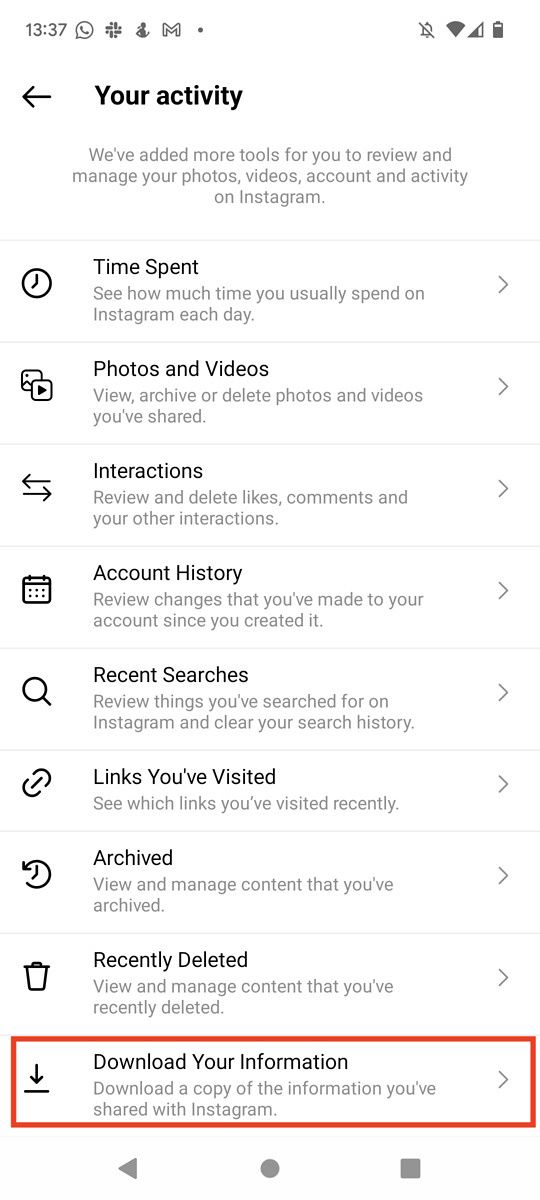The image depicts the settings menu on Instagram, featuring a detailed list of tools and options for managing your account. At the top of the menu is a left-pointing arrow icon, labeled "Your Activity." This section provides various tools to review and manage your photos, videos, account, and activity on Instagram. 

The menu items are listed as follows:

1. **Time Spent**: Tracks and displays the amount of time you spend on Instagram each day.
2. **Photos and Videos**: Allows you to view and manage your shared photos and videos.
3. **Interactions**: Shows your interactions within the app.
4. **Account History**: Details the changes and history of your account.
5. **Recent Searches**: Displays a log of your recent searches.
6. **Links You’ve Visited**: Lists the links you have visited.
7. **Archived**: Enables you to view and manage content that you’ve archived.
8. **Recently Deleted**: Contains items that you have recently deleted.
9. **Download Your Information**: At the very bottom, outlined in an orange rectangle, it offers you the option to download a copy of the information you’ve shared with Instagram.

Each menu item has a right-pointing arrow icon indicating that it can be selected for more details. The "Time Spent" section highlights your daily average usage of the app, whereas the "Archived" section allows you to view and manage photos and videos that you have archived.